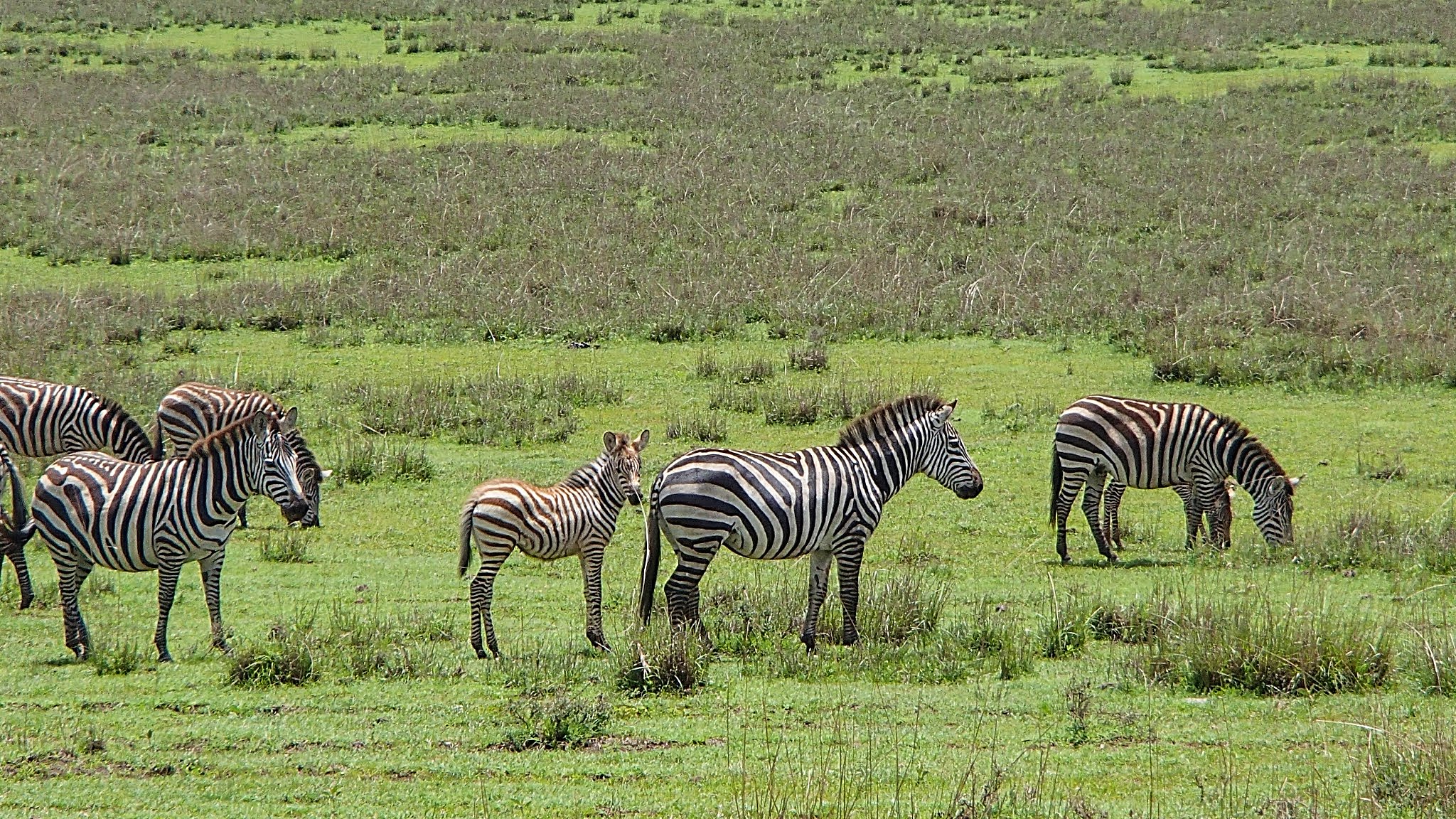This photograph captures a picturesque scene of a grassland teeming with a total of seven zebras. Among them, a smaller baby zebra with distinct light brown stripes stands out in the middle of the group, noticeably less than half the size of the surrounding adults, which have the characteristic black and white stripes. The adult zebras appear larger and more robust in comparison. The zebras are positioned in a variety of postures, some with heads lowered to graze on the mixed lengths of grass, while others stand upright, their heads raised. The field itself is a mix of short grass with interspersed patches of taller grass and small shrubs. The background of the photo reveals a striking contrast, where thicker, bushy grass appears in shades of green and slightly purplish hues. While most zebras align towards the left, the zebra at the center faces forward, and a partially visible zebra tail can be seen on the right edge, contributing to the symmetry and balance of this natural tableau.